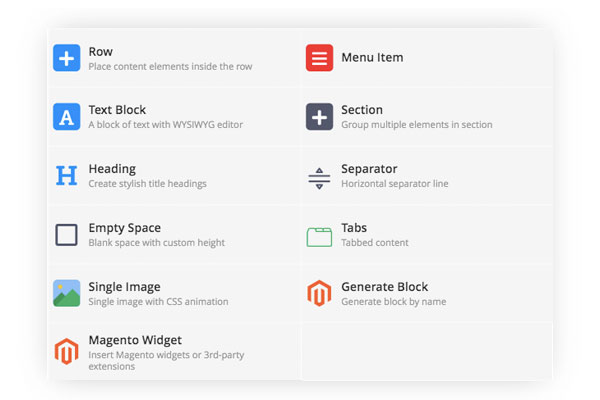The image is a detailed visual representation of a website layout editor, showcasing various content elements available for building a web page. 

In the top left-hand corner, the element labeled "Row" is highlighted in gray or black, with an accompanying description in gray that reads, "Place content elements inside the row." Directly below this, there is a "Text Block" element, described in gray as "A block of text with WYSIWYG editor."

Continuing down, the next element is "Heading" in black, followed by its description in gray: "Create stylish title headings." Below this is an "Empty Space" element in black, with a gray description that reads, "Blank space with custom height." Further down, "Single Image" is listed in black, accompanied by the text in gray: "Single image with CSS animation." 

At the bottom left, the element "Magento Widget" is highlighted in black, with its description in gray: "Insert Magento widgets or third-party extensions."

On the right-hand side of the page, the first item is "Menu Item" in black. Moving down, "Section" is listed in black with a gray description: "Group multiple elements in section." Below this is the "Separator" element in black, described in gray as "Horizontal separator line." 

Further down, the "Tabs" element appears in black, with a gray description: "Tabbed content." Finally, at the bottom, there is a "Generate Block" element in black, described in gray as "Generate block by name."

This comprehensive layout provides a clear guide to the various content blocks and their functionalities within the website editor.